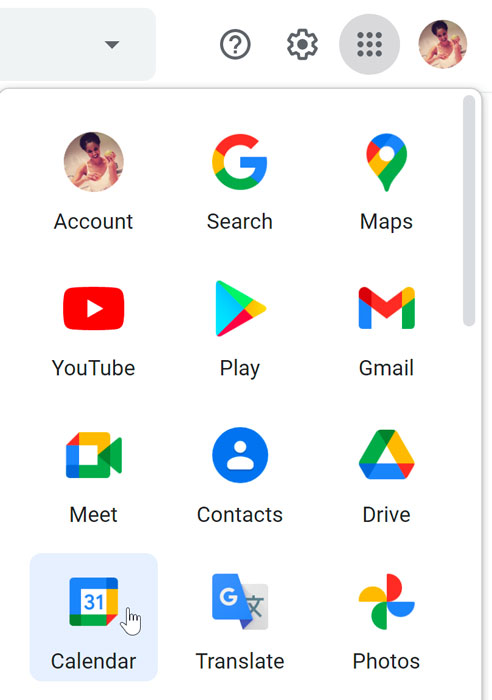This image is a screenshot likely taken from a smartphone. The interface primarily features various Google products arranged in a grid format. At the very top right corner, there is the profile photo of a woman with short, dark brown hair styled in a pixie cut. She is wearing a white tank top. 

To the left of the profile photo is a gray circle containing nine darker gray dots, resembling an app grid icon. Next to that on the left is an icon that looks like a gear, indicating settings, followed by a gray circle with a question mark, suggesting help or support. Further left is a very light gray square with an inverted triangle, indicating a drop-down menu.

The background of the image is white, and the main section displays three rows across and four rows down of various Google product icons, totaling twelve. Starting from the upper left, there is the user's account profile labelled "Account." The other icons featured are for Google services: Search, Maps, YouTube, Play, Gmail, Meet, Contacts, Drive, Calendar, Translate, and Photos. Each icon is distinct and representative of its respective service; for example, the Google Play icon is a colorful play button shape, and the Google Drive icon features three colors forming a triangular shape.